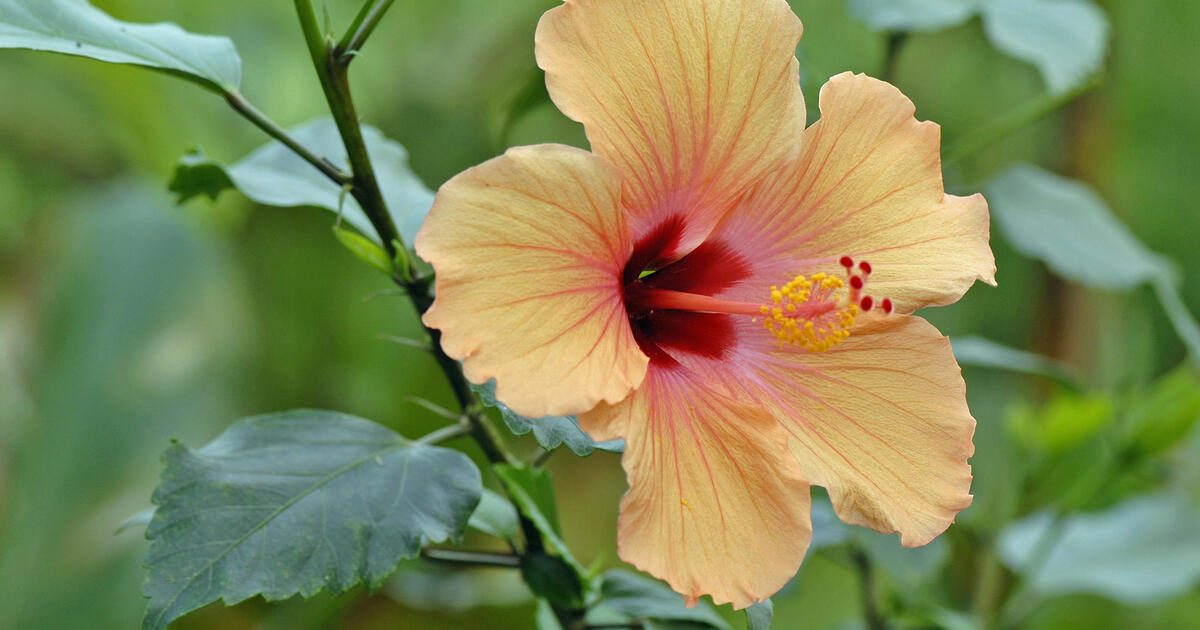This professional close-up photograph captures the intricate beauty of a hibiscus flower in exquisite detail. The flower features five slightly ruffled petals with a delicate light peach base color, adorned with vibrant pink veins that branch outward towards the edges. The petals' pink veins transition into a deep red at the flower's center, creating a striking focal point. Emerging from this center is a prominent red stigma, adorned with small yellow and slightly larger red dots at its tip. The hibiscus is attached to a green stem, which supports four or five broad, alternating leaves. The background is artistically blurred, showcasing subtle shapes of additional foliage and contributing to the vivid and colorful depiction of the flower.